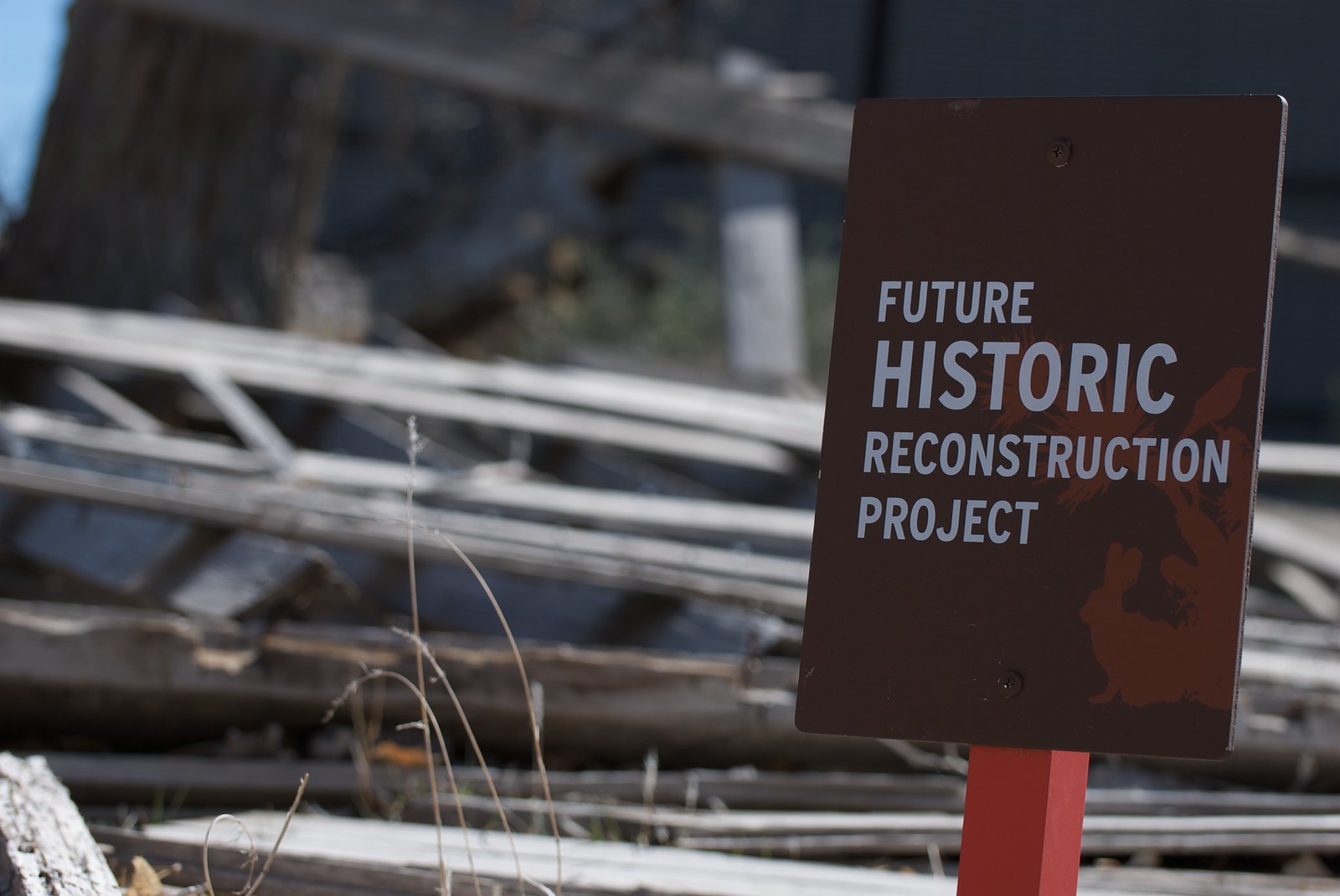The image, taken outdoors during daytime, captures a professionally made, vertical rectangular sign mounted on a prominent red post. The sign, dark brown in color, features white capital letters that announce "FUTURE HISTORIC RECONSTRUCTION PROJECT." Situated in the foreground are a few blades of tall, dry grass, while the background reveals a somewhat messy scene with logs, wooden debris, and what seem to be remnants of wood construction materials scattered on the ground. A tree and a larger structure partially obscured by overgrowth are visible in the distance. Adding a touch of intrigue, the bottom right corner of the sign displays a lighter brown silhouette of what appears to be a rabbit. A hint of blue sky peeks out from the upper left corner, setting the stage for an impending construction effort likely part of a historic district project.